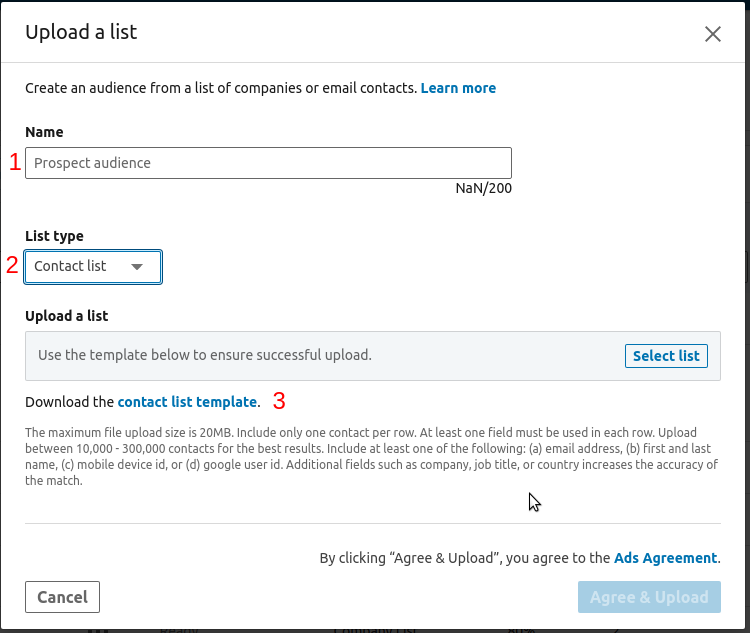The image depicts a digital interface for creating an audience from a list of companies or email contacts. The window instructs users to upload a list and fill out fields labeled "Name" and "Prospect Audience." The interface specifies a character limit of 200 characters for entries. Users must select a "Contact List" as the list type and follow a step-by-step guide to ensure successful uploads. An option to download a contact list template is available. Steps are numbered beside each action (1 for Name, 2 for List Type, 3 for Contact List Template). A green "Upload" button is prominently positioned in the bottom-right corner, indicating the final step in the process. This system appears designed to help users generate leads efficiently.